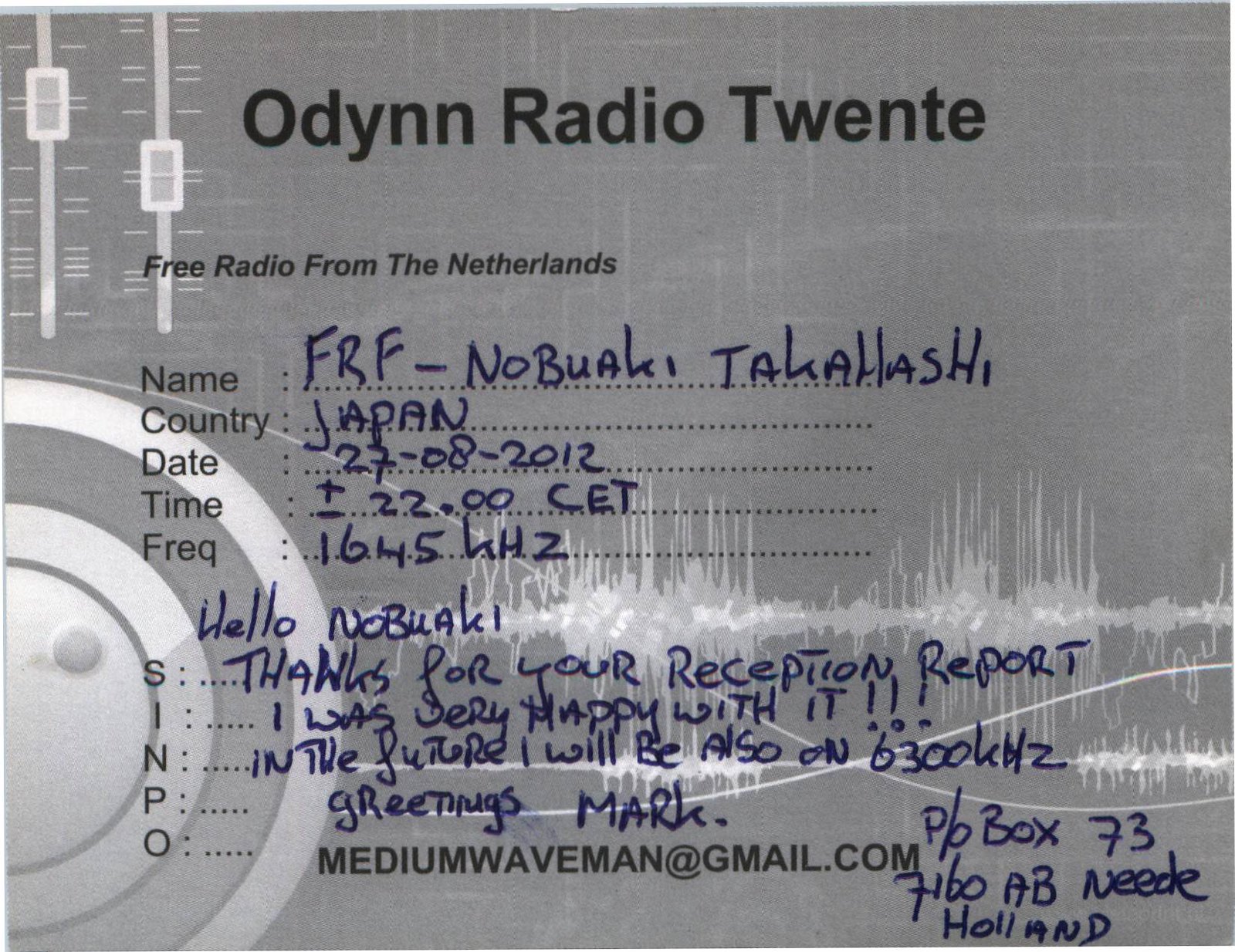The image depicts a card resembling a handwritten postcard or thank-you note, predominantly in black and white with gray shades. There's a detailed audio-themed background featuring what looks like waveform patterns, possibly representing a frequency, along with elements resembling headphones and knobs. 

At the top of the card, in black text, it reads "ODIN Radio 20" with "ODIN" spelled as "O-D-Y-N-N" and "20" as "T-W-E-N-T-E," followed by "Free Radio from the Netherlands." Below this, lines filled out in blue ink list "Name: FRF Nobukai Takahashi, Country: Japan, Date: 27-08-2012, Time: ±22.00 CET, Frequency: 1645 kHz, SINPO." 

A handwritten note addressed to Nobukai reads, "Hello Nobukai, thanks for your reception report. I was very happy with it. In the future, I will also be on 6300 kHz. Greetings, Mark." An email address, "mediumwaveman@gmail.com," is printed at the bottom, with a handwritten P.O. Box address to the lower right corner, "P.O. Box 73, 50 AB Need, Holland."

Overall, the image combines the structured look of a typed card with personalized handwritten elements, set against a background featuring audio design motifs.